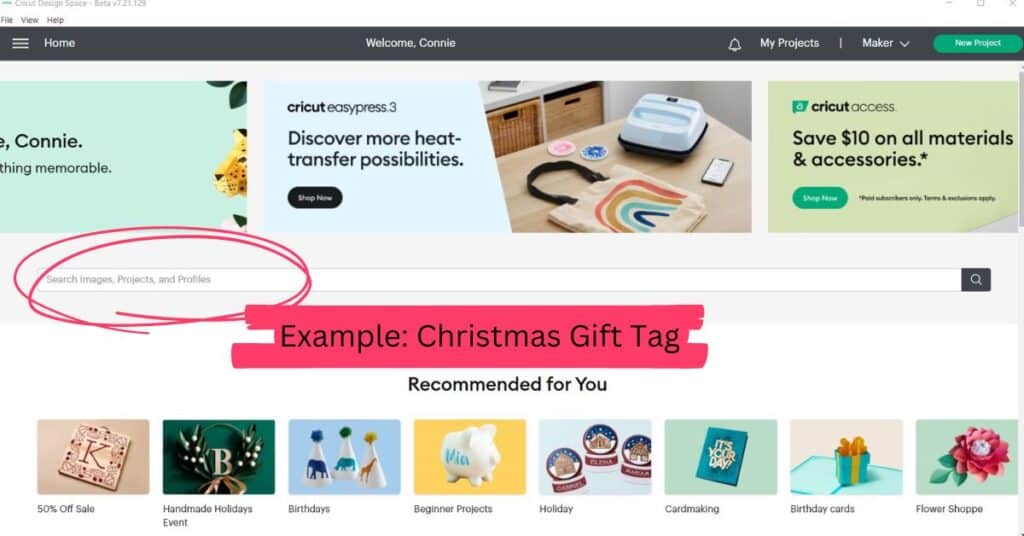This is a detailed and cleaned-up descriptive caption for the provided image:

---

The screenshot displays a web page dedicated to items primarily associated with cricket. In the top left corner, there are options labeled 'File,' 'View,' and 'Help.' Below, against a black background, is a bordered section with 'Home' on the left. Centrally located on the screen, a greeting reads 'Hello Connie' or 'Welcome Connie' next to a bell icon and the text 'My Projects.' At the top right, the phrase 'New Project' is highlighted in green.

To the left, there is a partially cropped image featuring the name 'Connie' and the phrase 'Thing Memorable' against a blue background, seemingly depicting part of a large cat's, possibly a cheetah's, head.

Dominating the center of the page is a large promotional image with the text 'Cricut EasyPress 3. Discover more heat transfer possibilities.' This is accompanied by an image of a Cricut machine and various crafting supplies. Adjacent to this, promotional text reads 'Cricut Access. Save $10 on all materials and accessories,' alongside a green 'Shop Now' button.

Below the promotion, a search bar highlighted with a red oval is visible, containing the placeholder text 'Search Images, Projects, and Profiles.' Under this, an image with a red background features the text 'Example Christmas Gift Tag,' followed by a section labelled 'Recommended for You.' This section displays eight images, each with captions: '50% Off Sale,' 'Handmade Holidays Event,' 'Birthdays,' 'Beginner Projects,' 'Holiday,' 'Card Making,' 'Birthday Cards,' and 'Flower Shop.'

---

This caption provides a coherent and detailed description of the web page screenshot, highlighting key sections and visual elements.